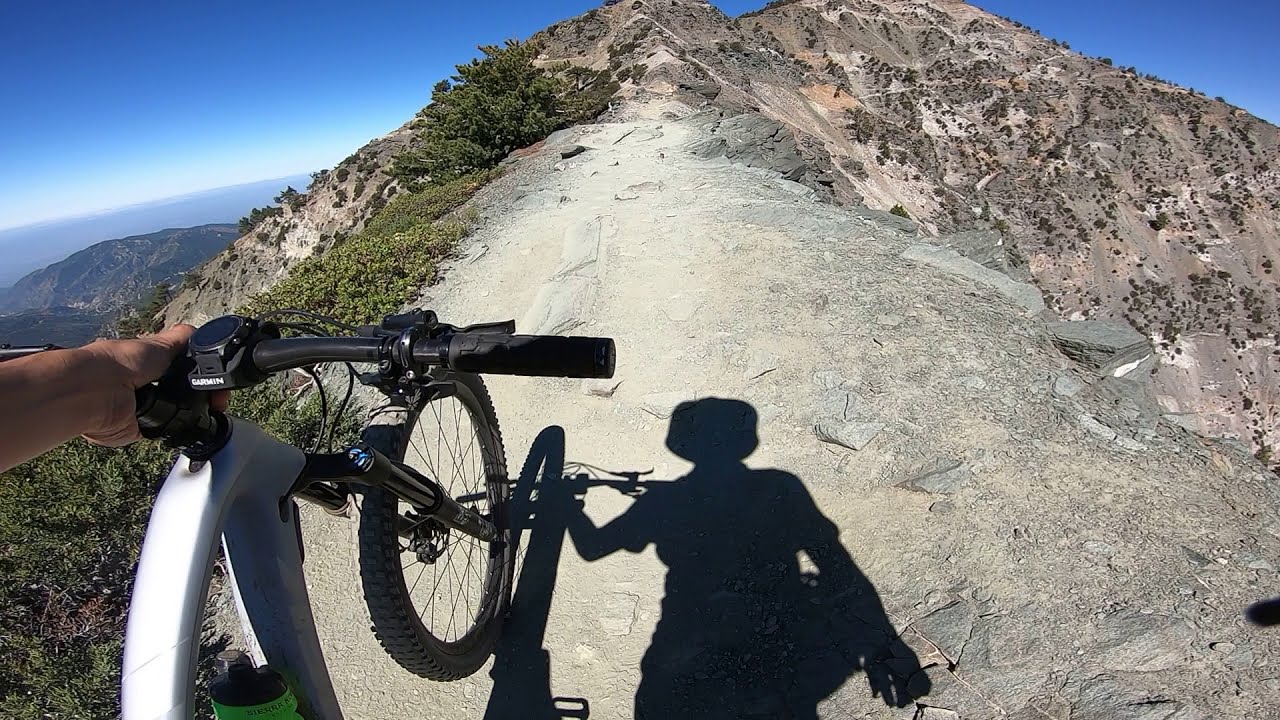The image captures a rugged, high-altitude mountainside with a horizontally-aligned rectangular composition. The foreground features a close-up of a person maneuvering a mountain bike along a steep, rocky incline. The bike, positioned on the left side of the frame, has a white frame with black handlebars and grips, and a mountain bike-style tire. A green water bottle is attached to the bike, and a singular hand can be seen gripping the left handlebar. The person's shadow is prominently cast against the smooth stone surface, indicating their stance as they climb. The rocky terrain transitions from light-colored stone near the viewer to more brown and jagged rocks further up. To the right of the incline, green plants and trees cling to the mountainside, while the distant background reveals additional lower mountain peaks. The sky above is a vibrant blue with a touch of white clouds scattered far off, hinting at the soaring altitude and expansive horizon. The top of the peak is just out of frame, leaving a sense of anticipation and adventure.